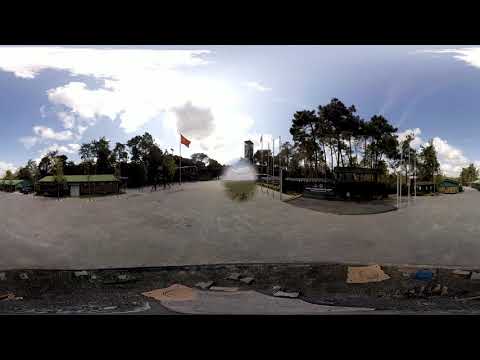This detailed exterior photo captures a bright, partly cloudy day in a parking lot or entryway to a park, viewed from a car window. The sky, punctuated by fluffy white clouds, hints at coming sunshine, promising a warm day ahead. Palm trees and other tall trees with lush, green foliage dot the background, while a flag, whose design isn't discernible, flutters from a flagpole. There are multiple buildings visible: to the left, a structure with brown walls, a white door, and a green roof, and further to the right, more buildings or homes. The overall scene exudes a sense of openness and tranquility, marred slightly by a small patch of garbage visible at the base of the image and a blurry dot that could be a water droplet on the camera lens. The image appears to be distorted, as if it were originally a panoramic shot flattened for viewing. The area provides several directional choices: moving forward into the park, turning left to explore, or heading right toward more buildings. The foreground includes a reflective surface likely from the car, enhancing the blurred effect. Despite minor imperfections, the inviting weather and open layout make it an ideal day to be out and about.